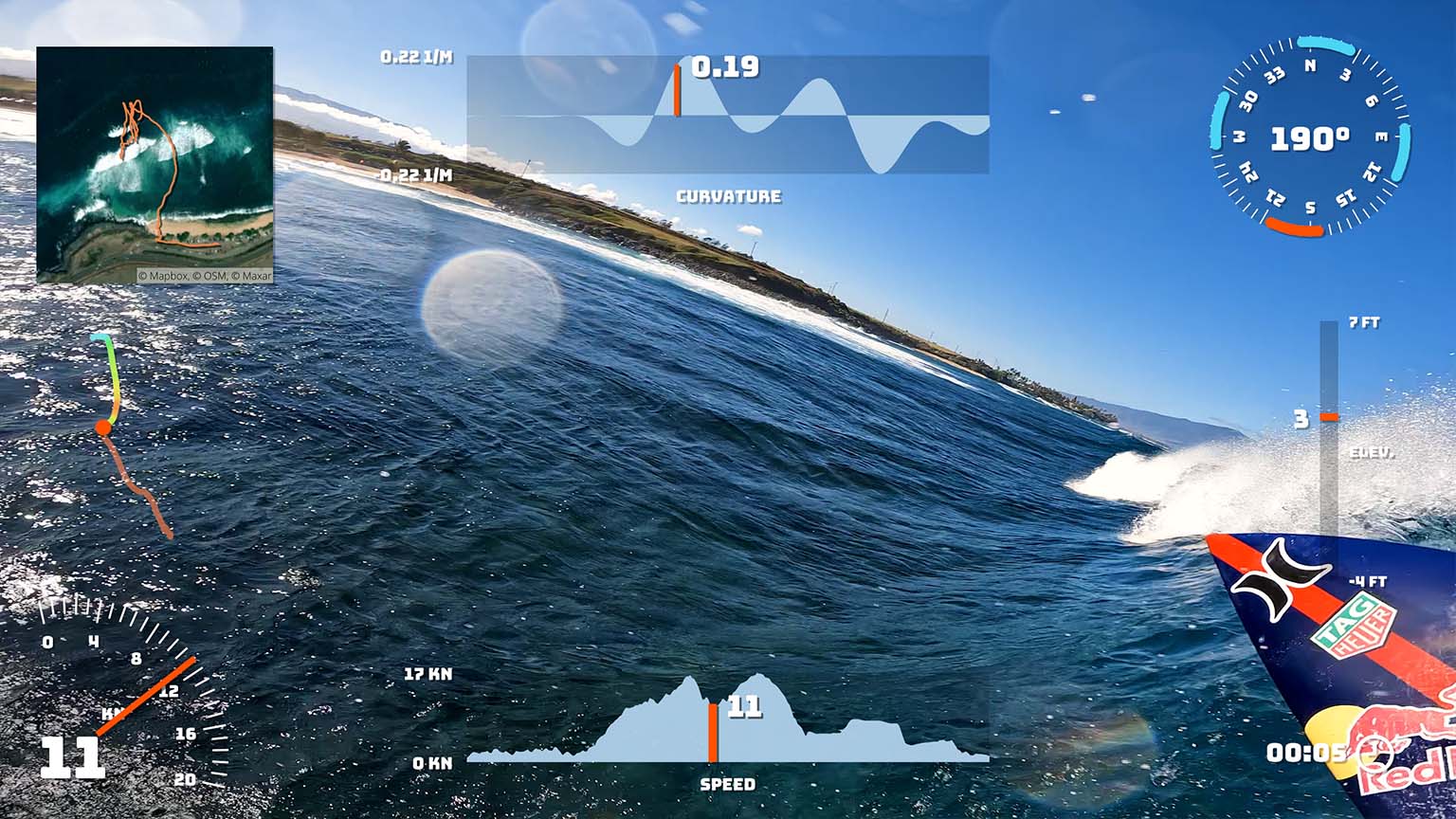This image captures a dynamic scene through a digital HUD, providing a comprehensive perspective likely from a GoPro attached to a surfer. The left side of the HUD depicts an overhead map view of a beach with an orange squiggle extending towards the water, indicating the location of the surfer. The lower left corner displays a speed indicator labeled at 11 km/h, which is visually represented by a red line in a wave-like graph at the center of the image. Adjacent to this, the left side also shows a bar graph with markers at 17 kn and 0 kn.

On the surfboard, inscribed with "Tag Hightower" and "Red Bull," there are two black C's facing away from one another, accompanied by a red line, set against a blue background. The elevation graph above this ranges from 4 to 7 feet, with the current elevation marked at 3 feet. The top right corner shows coordinates typically associated with a compass, set at 190 degrees, and another heading showing a 00.05 time stamp.

In the distance, an island lush with greenery is visible, contributing to the vibrant backdrop of the blue ocean and sky. Positioned on the right of the HUD is a chart displaying the wave height, highlighting a current measurement at 3 feet, suggesting the surfer is navigating a moderate wave. The overall scene suggests an active surfing session, with ample telemetry providing detailed real-time statistics of the surfer's performance and environment.